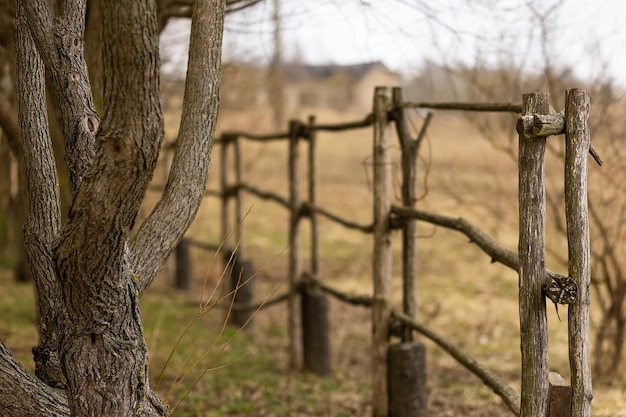The photograph depicts a rustic, outdoor scene featuring a handmade wooden fence and a tree. The fence, constructed from local tree branches, stretches from the right foreground to the left, gradually fading into the distance. In the foreground on the left, there's a small to medium-sized tree with numerous branches, showcasing the natural setting without any leaves, indicating a late fall or winter season. The fence appears aged and not very sturdy, with sections potentially held together by barbed wire or vine. At the base of the fence are wooden or possibly concrete posts that provide minimal support. The cloudy sky casts an even, diffused light over the scene, eliminating any harsh shadows. In the blurred background, beyond a large grassy field, stands a house with tan walls and a darker roof, adding to the rural atmosphere of the photograph.